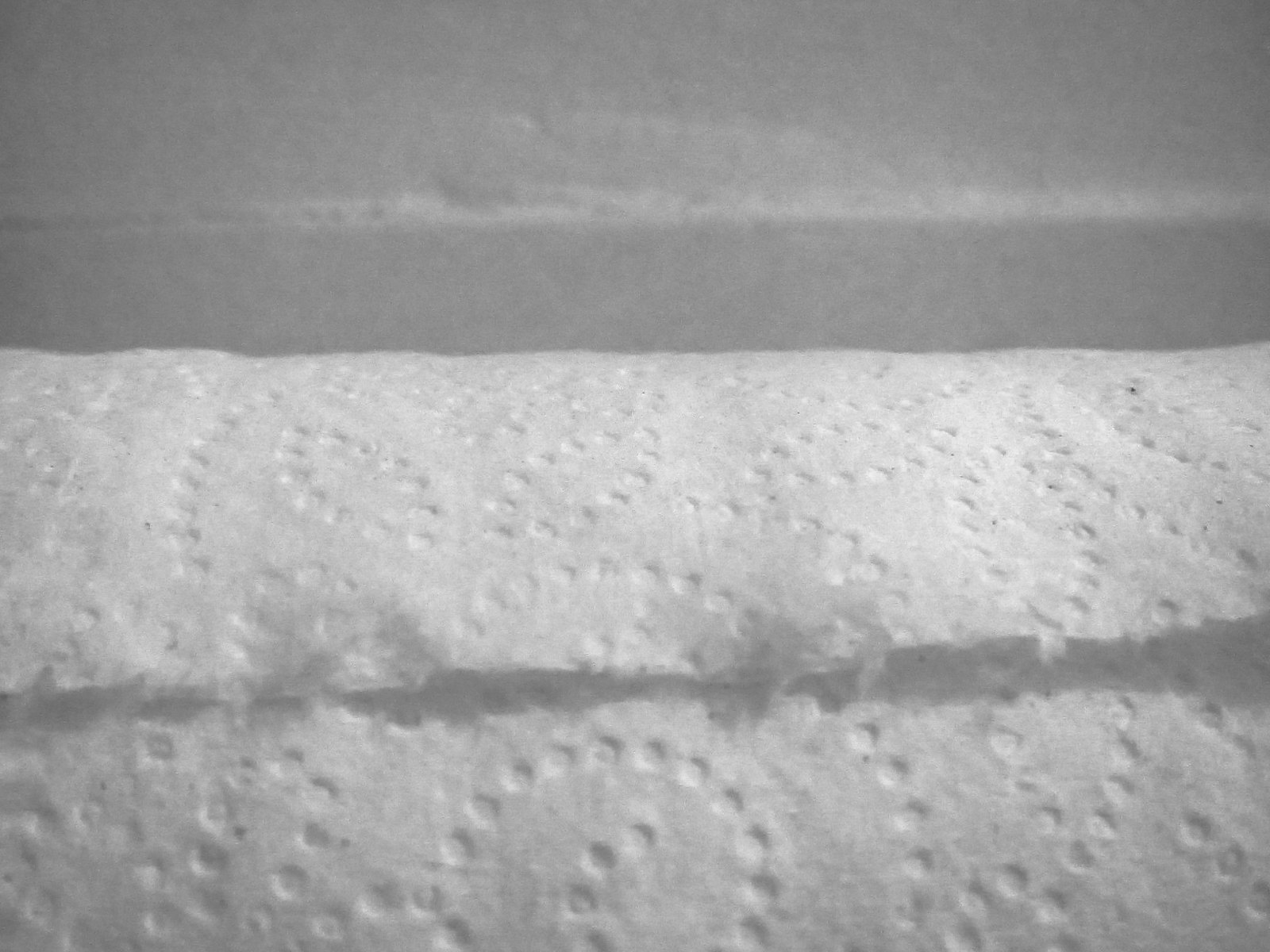This black and white image predominantly features a horizontally positioned, partially used roll of paper towels near the bottom of the frame. The roll extends from left to right, occupying much of the lower portion of the photo. The towel's texture and perforations are clearly visible, including detailed designs resembling punched holes, dots, and leaf-like patterns. The edge is frayed, indicating that a sheet has been torn off. Above the roll, the background is a blurred, gradient gray with streaks and patches of white, adding to the overall haziness. The setting appears to be indoors, possibly inside a cabinet, but specific details remain indistinguishable. There are no colors other than shades of gray and white, and the image lacks any text.